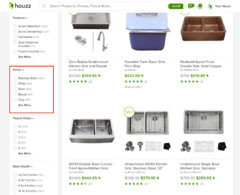This image depicts a screenshot of a website named Houzz, spelled H-O-U-Z-Z, which appears to be a platform selling various types of sinks. At the top of the page, the Houzz logo is prominently displayed. Centrally, there are six main listings, exhibiting an assortment of sink designs. The listings include stainless steel sinks and a unique golden sink. Some products feature a single basin, while others showcase double, side-by-side basins. One of the white sinks stands out with a contrasting blue accent. Adjacent to these listings, on the left sidebar, a highlighted section is demarcated by a red rectangle and line, drawing attention to specific filter options or categories. Green hyperlinks and star ratings are also visible throughout the image, indicating clickable elements and product ratings, respectively.